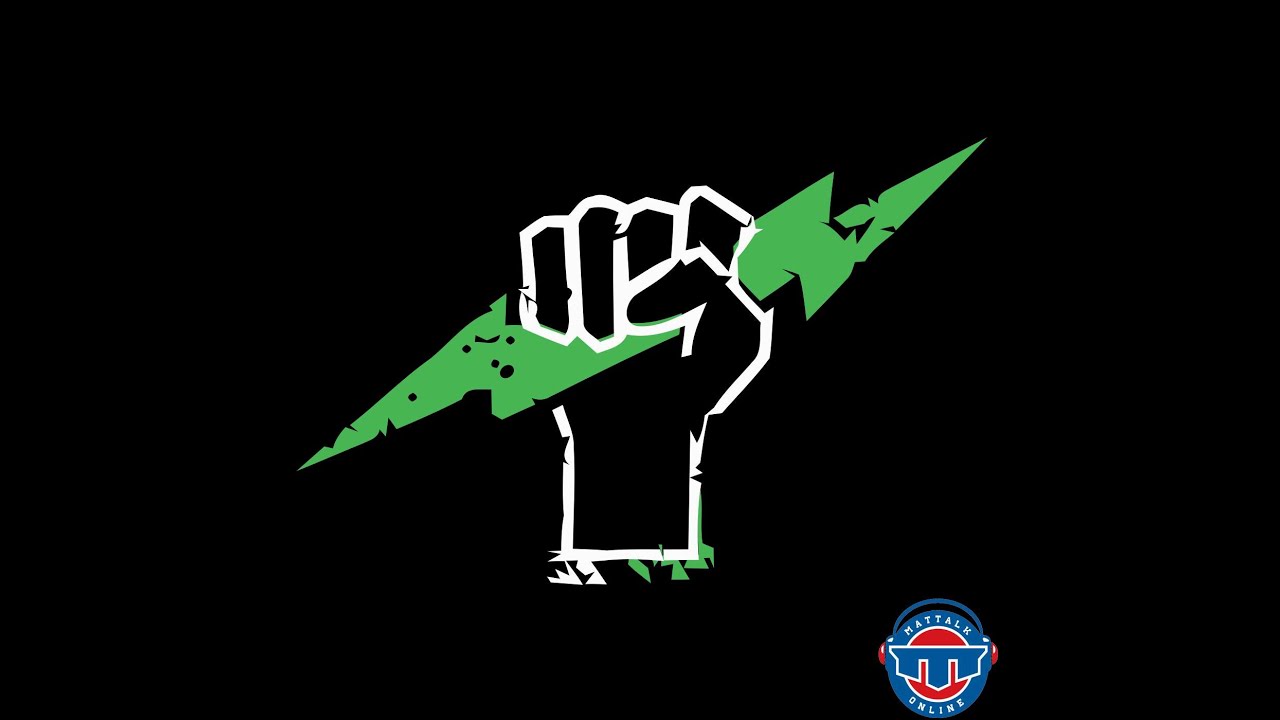The image features a striking logo centered on an all-black background. The prominent element in the middle is a white-outlined right-hand fist, with a thumb on the right side, gripping a lime-green lightning bolt. The bolt juts out sharply at both the top and bottom, creating a dynamic visual. The details are intricate, with the white outline of the fist and the lightning bolt exhibiting a grunge effect, characterized by small, triangular chips. Additionally, the interior of the fist and the areas within the lightning bolt show black, emphasizing the white outline. In the bottom right corner, there's another logo resembling a head wearing headphones. The head is depicted as a blue and red oval, with white text inscribed on it. The upper part of this text reads indistinctly, while the lower part clearly states "online." This small logo adds another layer of detail to the overall image.